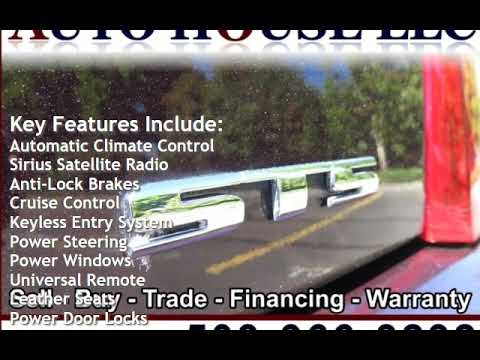The image appears to be a rectangular advertisement with thin black bars at the top and bottom. The top black bar partially obscures a heading, where only the bottom halves of the letters are visible; it likely reads "Auto House LLC." Dominating the center of the image is a photograph featuring the shiny, black tailgate of a vehicle, presumably a truck, with a silver STS emblem prominently displayed. Reflected in the vehicle's polished surface are trees, the sky, and a road. On the left side of the image, key features of the vehicle are listed in white block text, including automatic climate control, Sirius satellite radio, anti-lock brakes, cruise control, keyless entry system, power steering, power windows, universal remote, leather seats, and power door locks. Additional text at the bottom mentions "trade financing and warranty," although the bottom black bar partially obscures some text and a phone number on the bottom right corner. Overall, the advertisement highlights the vehicle's features, likely from a car dealership, emphasizing its many advanced amenities.